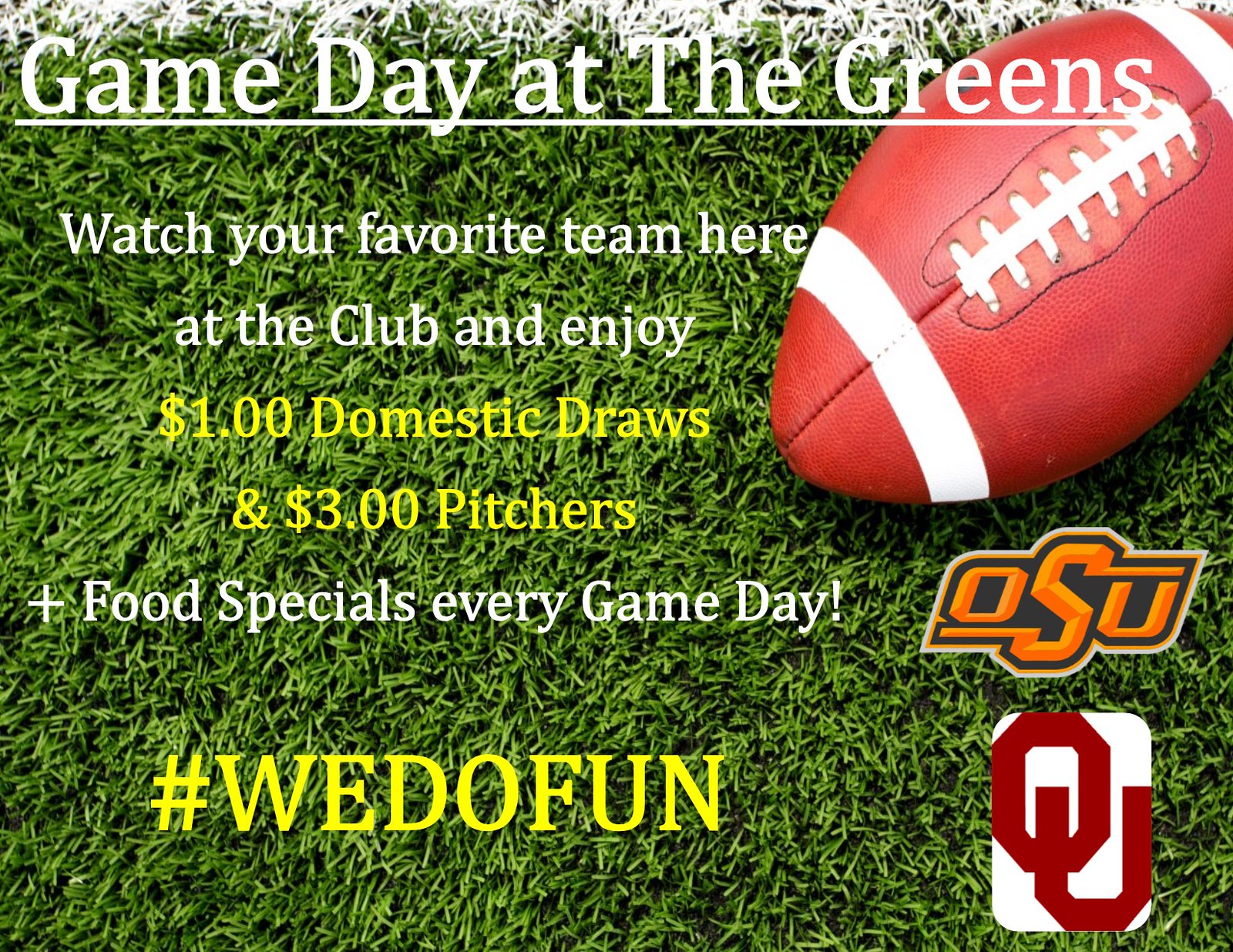The image is an advertisement for a college game day event at "The Greens." The background features green turf grass. At the top, in underlined Cambria font, it reads "Game Day at the Greens," followed by "Watch your favorite team here at the club and enjoy." The promotion text, also in Cambria font, highlights "$1 domestic draws and $3 pitchers" in bright yellow letters, and "plus food specials every game day" in white font. Towards the bottom, in bold Garamond font, it states "HASHTAG WE DO FUN" in big capital letters. On the bottom right corner, two logos are present: one for Ohio State University (OSU) and the other for the University of Oklahoma (OU), indicated by their respective colors and insignias. A reddish-colored football with white stripes and stitching is slanted from the middle up to the top right corner of the image, reinforcing the sports theme.